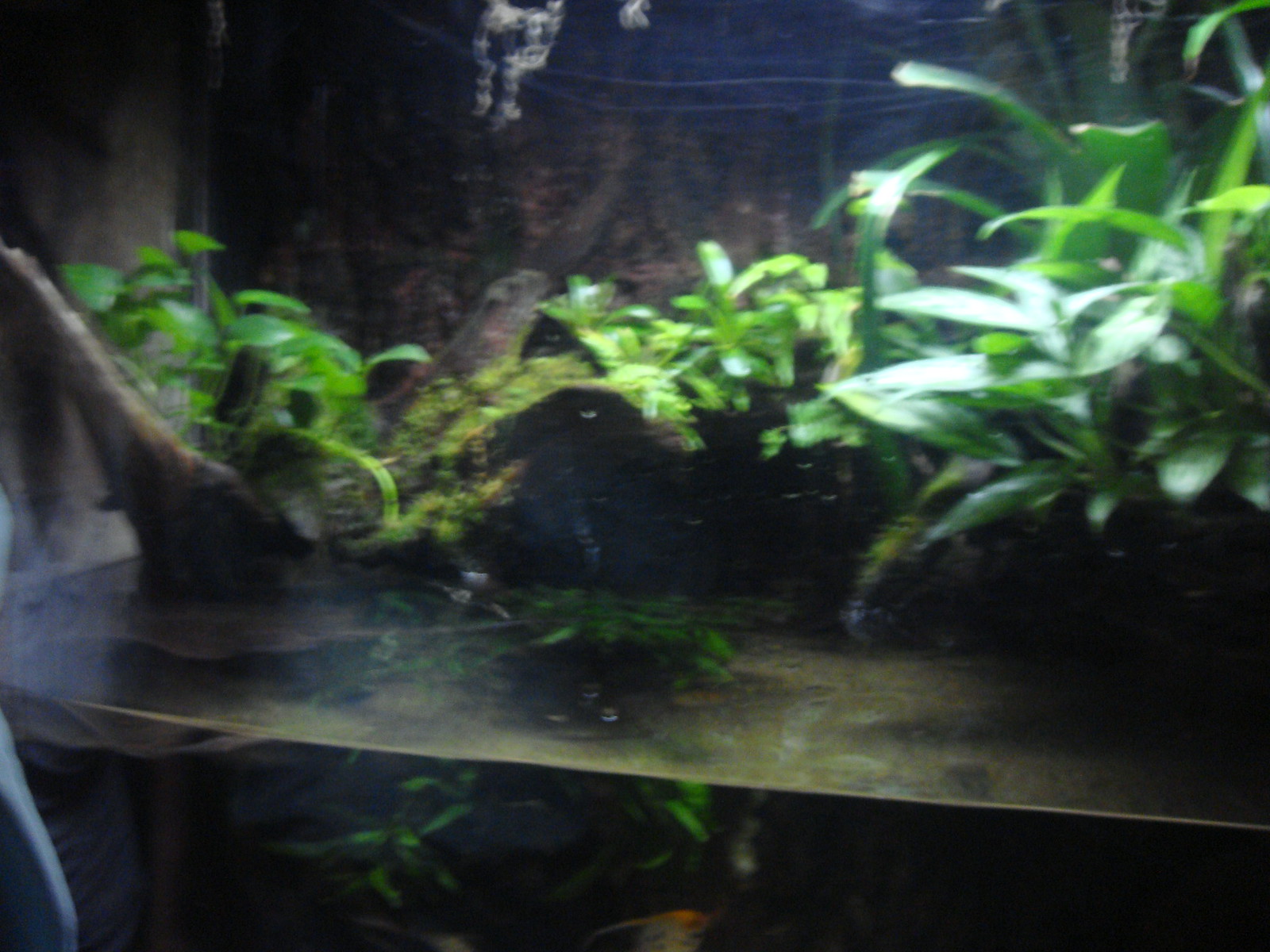The image features a slightly blurred scene of several small potted plants displayed on a brownish-gray stone or wood surface. The plants showcase a range of green leaves, varying in shape from long and thin to short and vine-like, with some extending past the table's edge and hanging below it. Under direct white light on the right side, the leaves appear bright green, while those towards the center and left are less illuminated but still visibly green. The backdrop is a very dark background, partially revealing a brown textured wall with hints of white light at the top. Additionally, there appears to be a cylindrical object in the background, splitting into two sections.